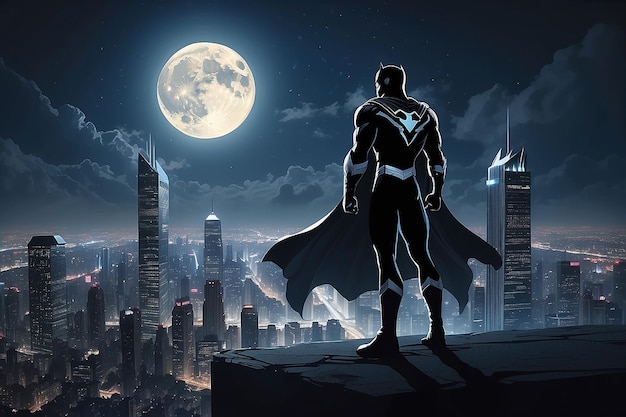The image is a detailed comic book-style illustration set at night. The background features a vast, dark sky in shades of bluish-black, dotted with hints of white stars and enveloped by gray clouds arching around a bright, prominent moon. Beneath this celestial scene stretches a sprawling cityscape of skyscrapers and lit-up streets, their lights twinkling like stars. In the foreground, on the right edge of the image, stands a figure unmistakably resembling Batman. Clad in a tight-fitting black outfit with silver accents, he wears a black cape with gray trim that billows dramatically, creating an eerie visual effect as it appears to be both in front of and behind him. Batman's pointed ears and iconic silhouette are instantly recognizable as he gazes out over the city's buildings from a high platform, creating a striking juxtaposition of the brooding character against the luminous urban night.